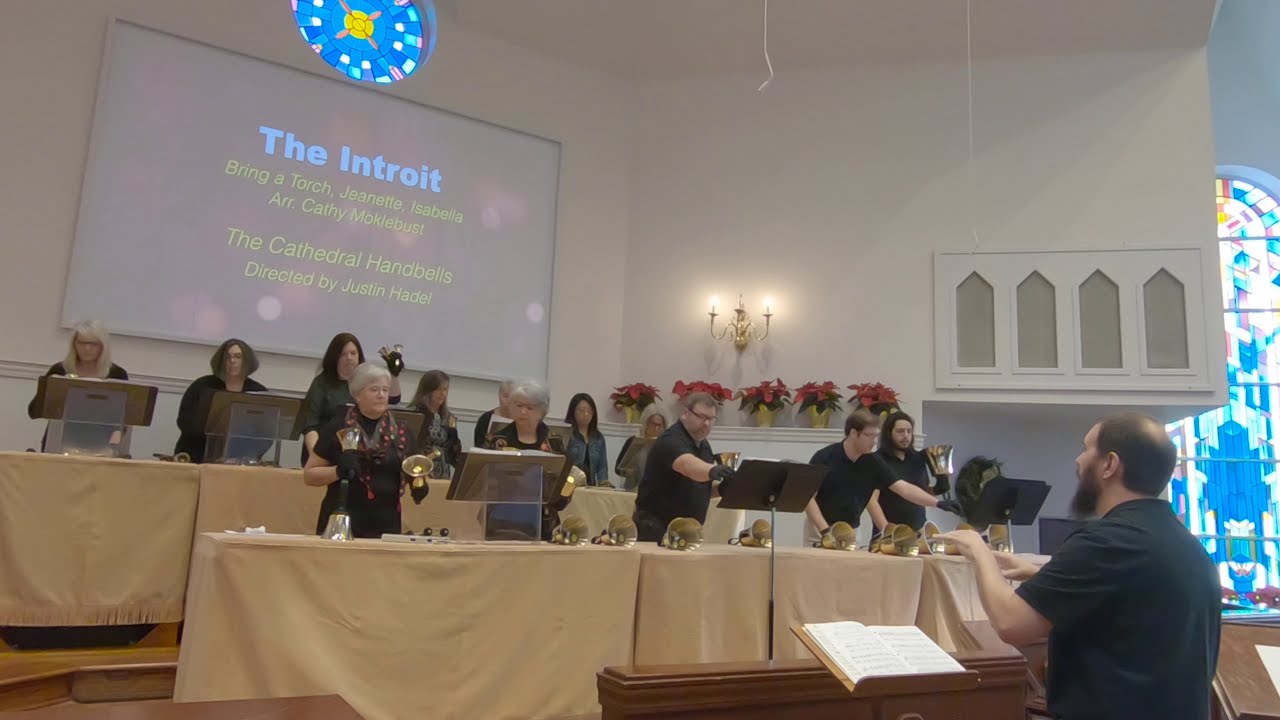This photograph captures a church service featuring a group of men and women standing at two tables, both covered with beige cloths, and adorned with brass handbells. Most of the participants, particularly the men, wear black short-sleeve shirts. The setting includes a round stained-glass window at the top left and additional stained-glass windows to the right. A large screen on the left displays the text: "The Introit" in white, followed by "Bring a Torch, Jeanette, Isabella" in yellow, and then lists "R, Cathy, Mucklebust" alongside "The Cathedral Handbells directed by Justin Hadel." The scene is further embellished with a red poinsettia plant arrangement and an electric candlestick with two lights affixed to the white walls. At the bottom right, a bearded man in a black shirt appears to be directing the ensemble, who are focused on stands holding music or papers.